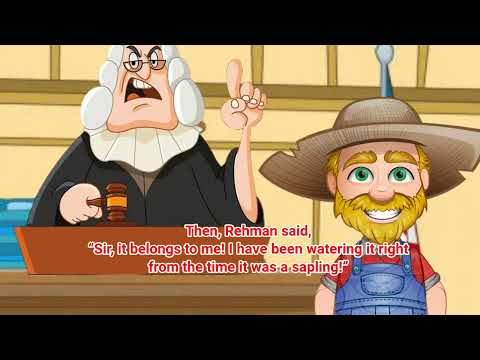The image is a vibrant, cartoon-style illustration that seems to be a screenshot from a children's nursery rhyme video. It depicts two smiling farmers standing side by side against a picturesque backdrop of rolling green grass, a lush green tree, and distant mountains under a blue sky dotted with puffy white clouds. The farmer on the left is a younger man with short brown hair, green eyes, and a tan straw hat. He is dressed in blue denim bib overalls and a green short-sleeved shirt with the sleeves rolled up above his elbows. The farmer on the right, an older man, sports a heavy, golden yellow beard and green eyes. He is wearing a darker, worn-out tan straw hat, blue denim bib overalls, and a red shirt. The caption in red font with a white outline at the bottom of the image reads, "There lived two farmers named Abu and Raymond in the kingdom of Emperor Akbar. They both were neighbors." The overall scene is warm and colorful, featuring various shades of green, blue, red, yellow, and tan, enhancing the playful, friendly atmosphere typical of children's content.